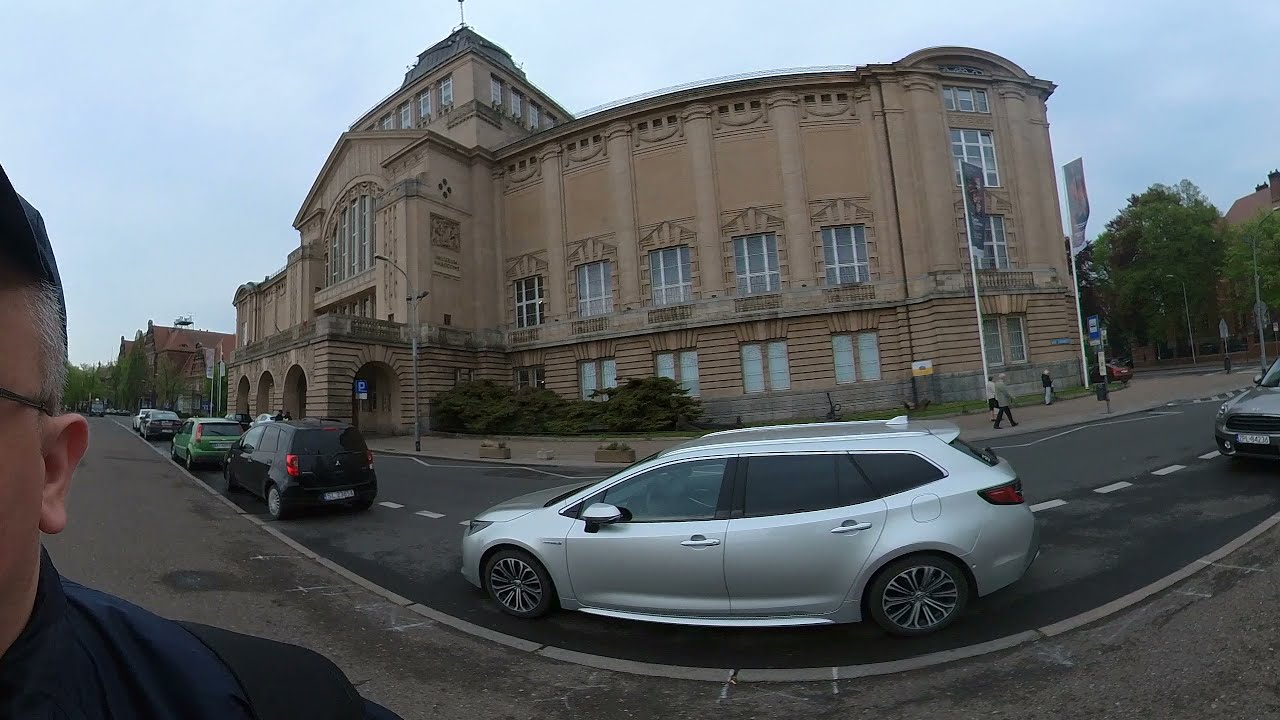A detailed image caption combining the repeated and shared details is:

A silver station wagon with tinted back windows and silver rims is parked on a concrete-colored curb in front of a large, brown building that resembles a courthouse or university. The building is three stories high with covered windows on the bottom level, an arched tall window above the entranceway, and a sharp-pointed architectural feature at the top. The entrance is made up of bricks and circular archways, with white poles possibly indicating flags or advertisements nearby. The sidewalk next to the curb has water stains and is light brown in color. A black minivan is parked in front of the silver car, followed by a green car and two other indistinct cars. Behind the silver station wagon is a darker gray vehicle with a white license plate. The sky in the background is very light blue with some haziness, and the clouds vary from light to dark. People are walking towards the right, one individual almost out of the picture on the far left, with visible details including a dark blue shirt, a cap, and glasses. The scene includes elements like trees, lampposts, and additional buildings, enhancing the setting's university-like appearance with students walking around.